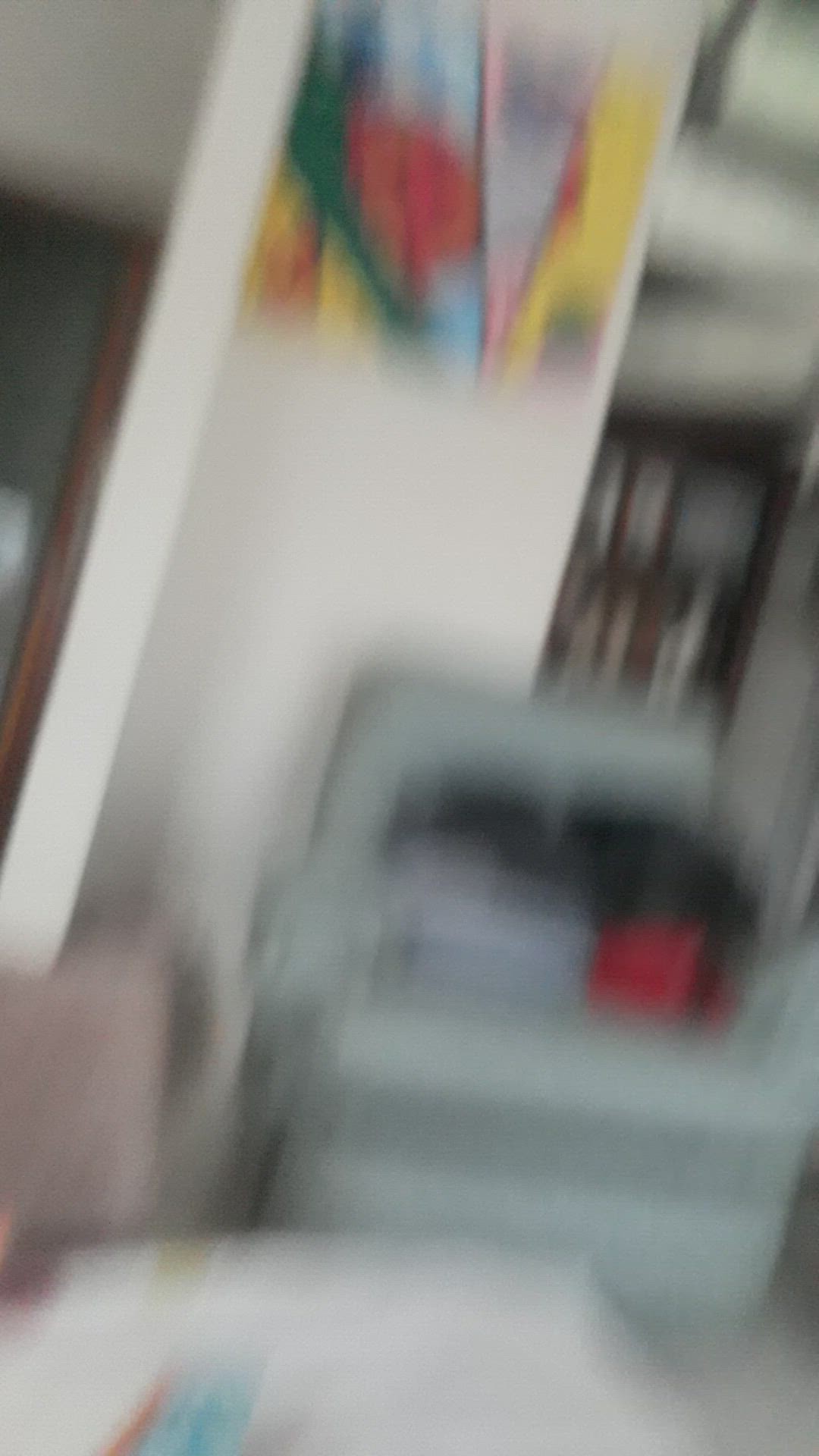This image portrays a slightly blurry view of a cozy living room. Central to the room is a prominent column adorned with an abstract painting. The painting is characterized by vibrant shades of green, orange, red, blue, yellow, and pink, sectioned by bold black lines that seem to have been drawn with a marker, creating a striking geometric composition. Below the painting, there is a plush, bluish recliner or single love seat, which is topped with various objects including blue and red items. In the background, a bookcase with a wooden frame is visible, adding a touch of warmth and homeliness to the scene. Additional black objects are scattered around, contributing to the room's lived-in feel.